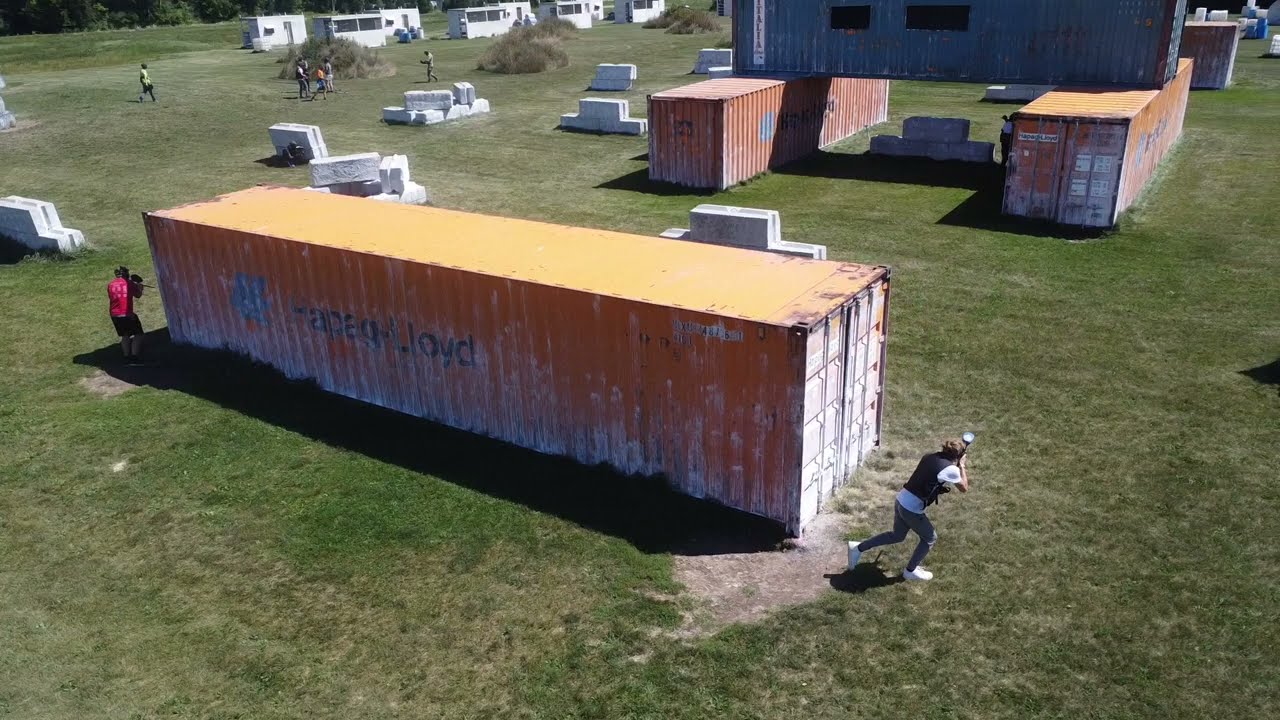This color photograph, captured by a drone in landscape orientation, provides a detailed aerial view of an outdoor paintball game in progress on a large, grassy field. The scene is primarily centered around an orange storage container positioned toward the center left of the photograph. This container exhibits numerous white paint streaks, indicative of its use as a paintball obstacle.

In the middle of the image, a man in a red shirt and dark shorts, equipped with a paintball gun and mask, peeks around the corner of this orange container. Directly to the right, another player in a white shirt, black vest, gray pants, and white sneakers stands poised with a paintball gun. They are engaged in the game, utilizing the container for cover.

Further into the field, three additional storage containers are strategically stacked to form a bridge-like structure – with two red containers on the bottom and a blue one placed perpendicularly on top. The field features an assortment of other obstacles, including white bunkers and large cinder block barriers scattered around, enhancing the strategic complexity of the game.

In the backdrop, there are several small white structures and a number of individuals standing on the sidelines, either observing the game or waiting for their turn to play. The photograph is rich with colors such as green from the grass, brown patches of dead grass, and bright hues from the various containers and participants' outfits, all bathed in daylight, suggesting midday activity on a dynamic paintball course.